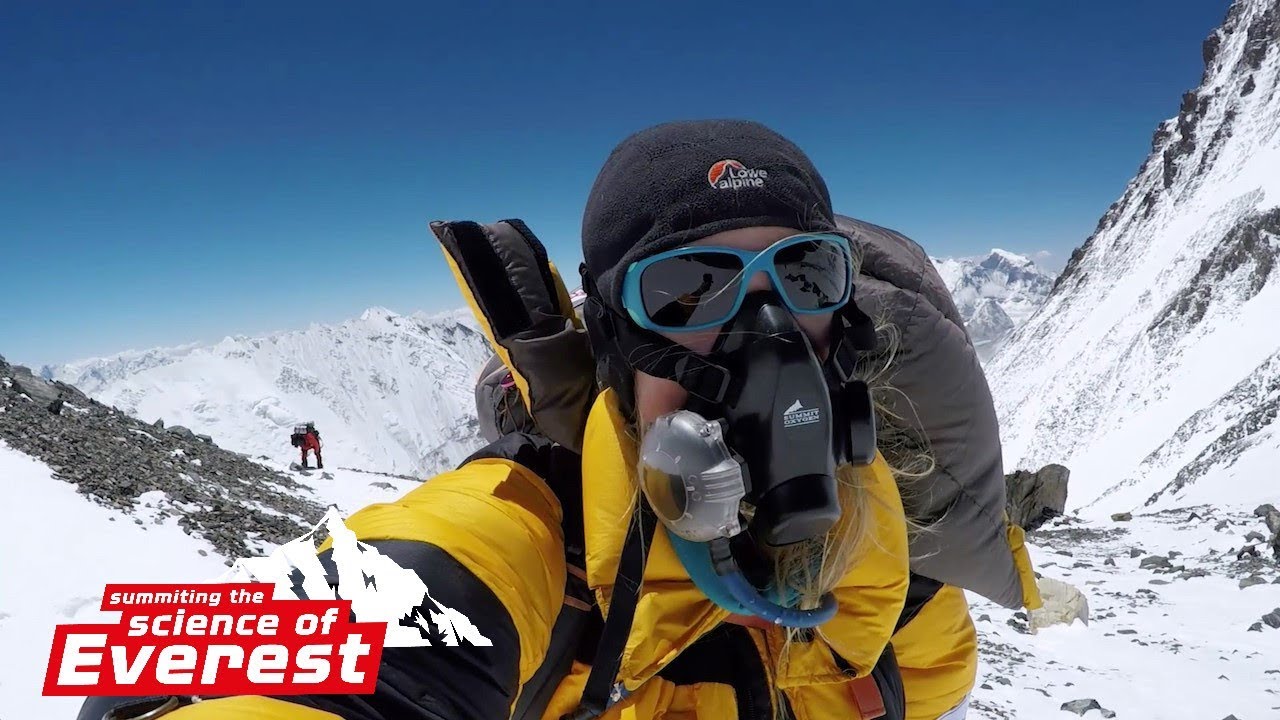A breathtaking photograph captures the stark beauty of a high-altitude, outdoor setting on what is likely Mount Everest. Dominating the center, a mountain hiker clad in a striking yellow parka with black accents stands resolute against a backdrop of snow-covered peaks. The hiker's face is obscured by a black breathing mask featuring a clear, circular component on the right side and a blue hose running along the bottom, indicating the challenging altitude. The hiker sports a black fleece cap from which tufts of hair escape, alongside blue-rimmed sunglasses that shield their eyes from the glaring snow. A large black backpack hints at the rigors of the trek. The deep, cloudless blue sky fades subtly into a lighter hue near the horizon, likely from the radiant reflection off the snowy slopes. 

To the left of the main subject, jagged rock formations peak through the snow, and a distant figure, small against the grand landscape, looks upward, underscoring the human scale against Everest's vastness. In the lower left corner, a red rectangular block with white text reads "Summiting the Science of Everest," next to a simplistic drawing of a white mountain, reinforcing the scene's location and the endeavor's scientific ambition. The image captures not only the climber’s equipped determination but also the awe-inspiring, unblemished expanse of one of the world’s highest and most treacherous peaks.